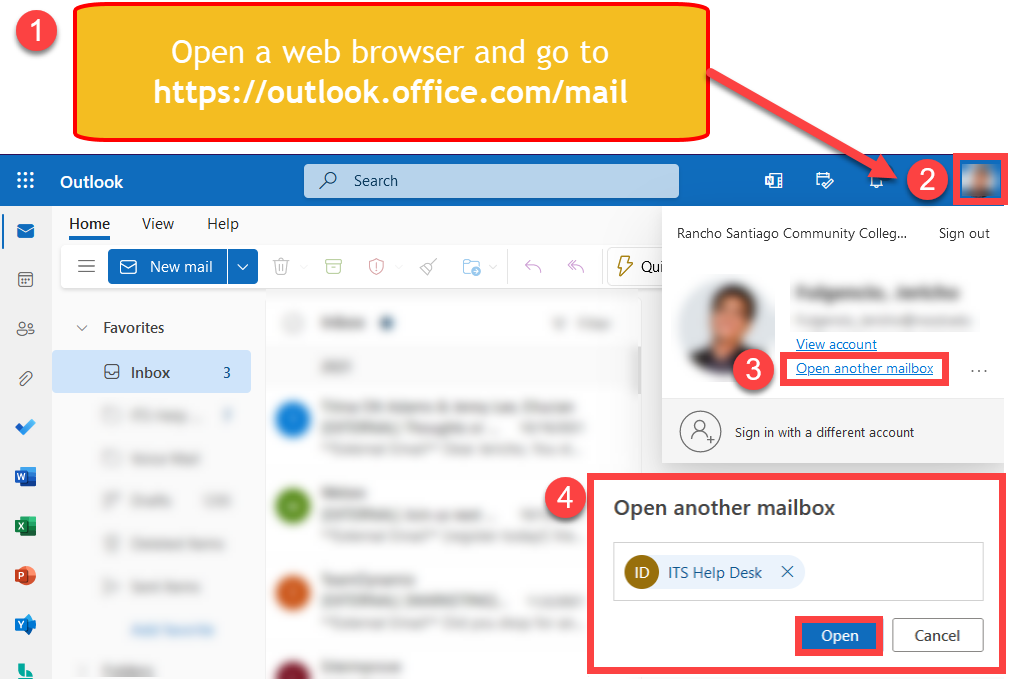This instructional image provides a detailed visual guide with steps on how to access and open a web browser to sign in to a specific website. Below is the cleaned and detailed description of the image.

1. In the top-left corner, there is a red circle labeled "1" positioned next to a large yellow block with a red frame around it. Inside this block, white text instructs the user to open a web browser and navigate to "https://outlook.office.com/mail".
2. A red arrow extends from the yellow block, guiding the viewer to the next step numbered "2". This step is indicated by a red rectangular border, suggesting the location for entering login credentials on the sign-in page.
3. The third step, labeled with a red circle and the number "3", is located nearby and corresponds to another action, namely opening a different mailbox.
4. Finally, step four, indicated by a red circle labeled "4", shows a white pop-up box associated with accessing another mailbox. Within this pop-up box, the text reads "ITS Helpdesk", and two buttons are visible: one labeled "Open" and the other "Cancel".

This detailed step-by-step visual guide effectively covers the process from opening the specified website to managing mailboxes and accessing assistance.